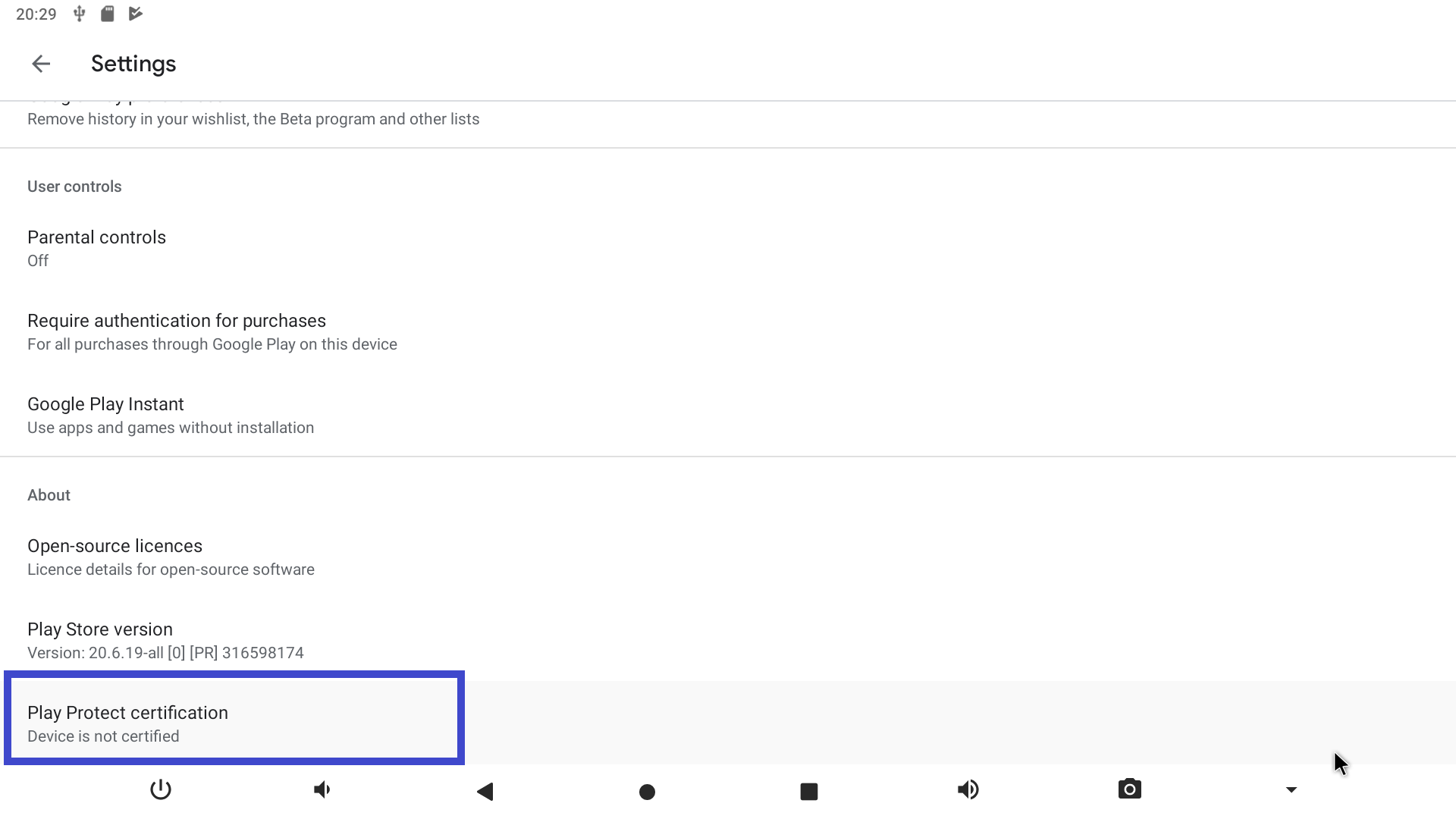This image is a screenshot captured from a cell phone or tablet, displaying a portion of the Google Play Store settings menu. At the top, the year "2029" is clearly visible along with an icon of a memory card and a triangle featuring a check mark inside. Below these icons, there is an arrow pointing to the left, and slightly to the right in bold print, the word "Settings" is prominently displayed with a capital "S."

A horizontal line follows these elements, with a partially cut-off line of text underneath. This text reads, "Remove history in your wish list, the beta program, and other lists," with "Beta" capitalized. 

Further down, the menu item "User Controls" appears, with "User" capitalized. This is followed by "Parental Controls" in a larger font and in all capital letters, and beneath this, the status "Off" is indicated. 

Next, the screen displays "Require authentication for purchases," specifying that authentication is needed "for all purchases through Google Play on this device." 

Further down, "Google Play Instant" is mentioned, offering the option to use apps and games without installation. Another horizontal line follows.

Below this line, "About" is listed, and underneath it reads, "Open source licenses," detailing "license details for open source software." Finally, the version information for the Play Store is presented as "Version 20.6.19-all [0] [PR] 316598174."

At the bottom of the screen, a blue rectangle contains the text "Play Protect certification," immediately followed by the status "Device is not certified."